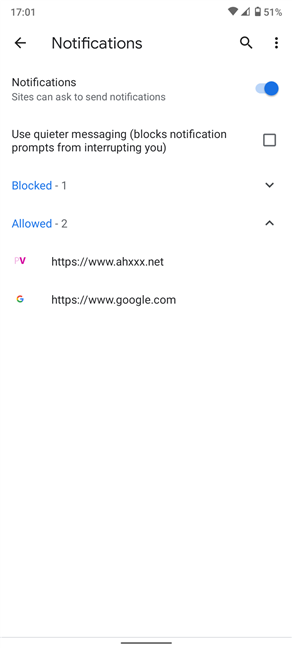Screenshot from a smartphone displaying the notification settings interface:

- **Top Bar:**
  - Upper left-hand corner: The time is displayed as "17:01".
  - Upper right-hand corner: Icons indicating the status of the fan, a triangle (possibly network status), and the battery at 51%.

- **Navigation Bar:**
  - Left side: A left-pointing arrow with the label "Notifications".
  - Right side: A search icon followed by three vertical black dots representing a menu.

- **Settings Section:**
  - Main title in smaller text: "Notifications".
  - Subtext in gray: "Sites can ask to send notifications".
  - Toggle switch: Light blue switch with a dark blue circle, likely representing an ON position.

- **Quieter Messaging Feature:**
  - Text: "Use quieter messaging (blocks notification prompts from interrupting you)".
  - Checkbox: Unchecked, adjacent to the quieter messaging description.
  
- **Notification Permissions:**
  - Labels: "Blocked" in blue with the number "1" next to an incomplete triangle pointing downward, and "Allowed" in blue with the number "2" next to an upward-pointing arrow.

- **List of Sites:**
  - First site: Icon labeled "PV" next to the URL "https://www.ahxxx.net".
  - Second site: Google icon next to the URL "https://www.google.com".